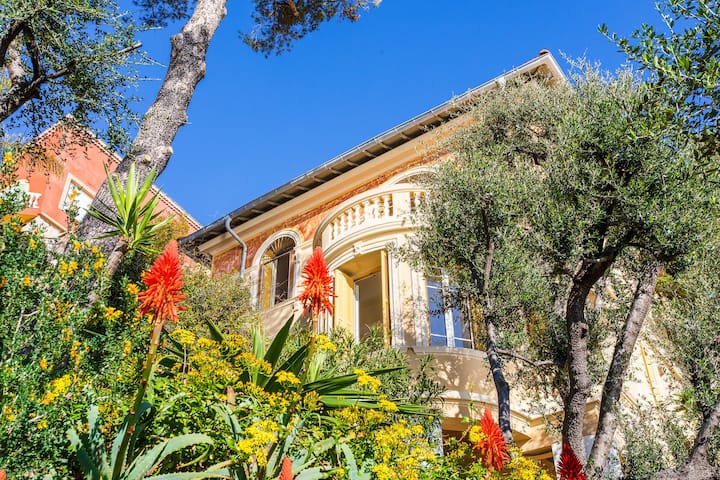This outdoor daytime photograph captures the upward viewpoint of someone kneeling to take a shot of a brick building adorned with white arches and a rounded, ball-front type window. Above this window is a decorative balustrade that likely supports a balcony. The gutter is visible on the underside of the roof. Adjacent to it, a taller brick building can be seen.

In the foreground, vibrant yellow and red flowers blossom, the red ones featuring triangular shapes. To the left of the building stands a tall tree with a long, leafless trunk that reaches up to the top of the image. On the right, a smaller tree with three or four branches exhibits scrub-like green leaves.

The building itself is a light brown or tan shade, casting a neutral contrast against the vivid plant life. Despite being partially obscured by the dense array of flowers and foliage that covers around 60% of the image, the building’s architectural details, including one arched window set outward and two flat arched windows, stand out. Some windows appear to be open. The clear, bright blue sky accentuates the tranquil yet dynamic outdoor setting, making the scene feel both lively and serene.